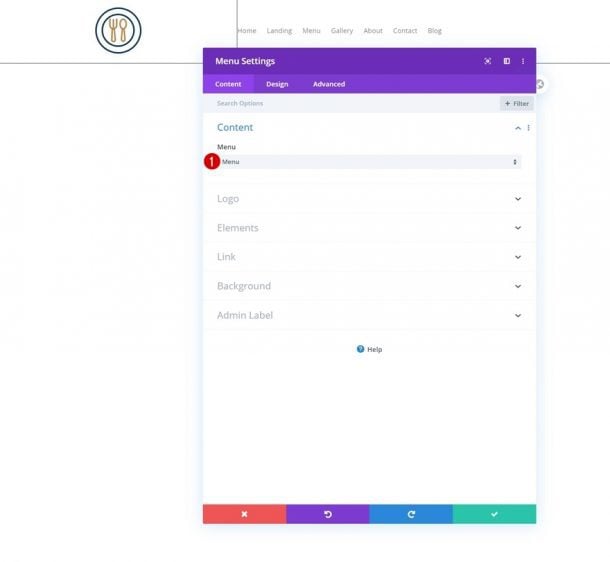Screenshot Description: 

The image is a screenshot of a website featuring a pop-up menu interface. The website itself has a minimalist design with a white background. In the upper left corner of the website, there is a simple icon depicting a plate with a red fork and knife on it. Adjacent to this icon on the right, there are various website navigation options listed in a gray font. The options include Home, Landing, Menu, Gallery, About, Contact, and Blog. However, due to the blurry quality of the screenshot, the text appears somewhat indistinct.

Dominating the center of the screenshot is the pop-up menu, which obscures most of the web page behind it. The pop-up menu consists of several sections and interface elements:

1. At the very top of the pop-up, there is a blue bar with white text. The left side of the bar displays "Menu Settings" while the right side features a small "X" icon which allows users to close the pop-up menu.
2. Below this is a lighter blue bar, also with white text, displaying three options: "Content," "Design," and "Advanced." The "Content" section is currently selected.
3. Within the selected "Content" section, there is a white window displaying various controls and information. The top of this window includes a gray bar with the text "Search Options" and a gray button labeled "Filter."
4. Underneath this, in black font, the word "Content" appears again, followed by "Menu." The "Menu" option has been clicked, and it is marked with a red badge containing the number "1" in white, indicating some form of notification or update.

Despite the low quality of the screenshot, the essential elements of the web page and the pop-up menu are discernible.